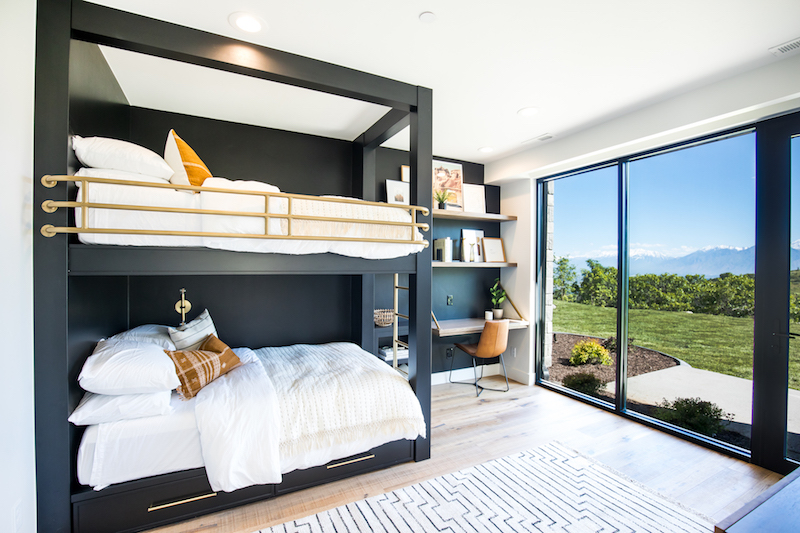This image showcases a modern and upscale bedroom in landscape layout. Dominating the left side are black-framed bunk beds with brass railings and a brass ladder at the foot. The beds are dressed in white bedding with plush pillows and comforters. On the floor lies a light wood floor, partly covered by a white rug with blue stripes.

A sleek white desk with a contemporary tan leather chair and a small plant is tucked into the back corner, between the sliding glass doors and the bunk beds. Above the desk, two shelves display various pictures. The large sliding glass doors on the right side reveal a scenic outdoor view, featuring a clear blue sky, distant mountain ranges, green grass, trees, mulch areas, and plants.

The room also includes a section of a stairwell leading up to the second level of the bunk beds and is characterized by a black wall that provides a contrast to the overall white and wood theme. This detailed setup exudes a contemporary and cozy atmosphere, possibly suggesting a space within a high-end Airbnb or hostel.